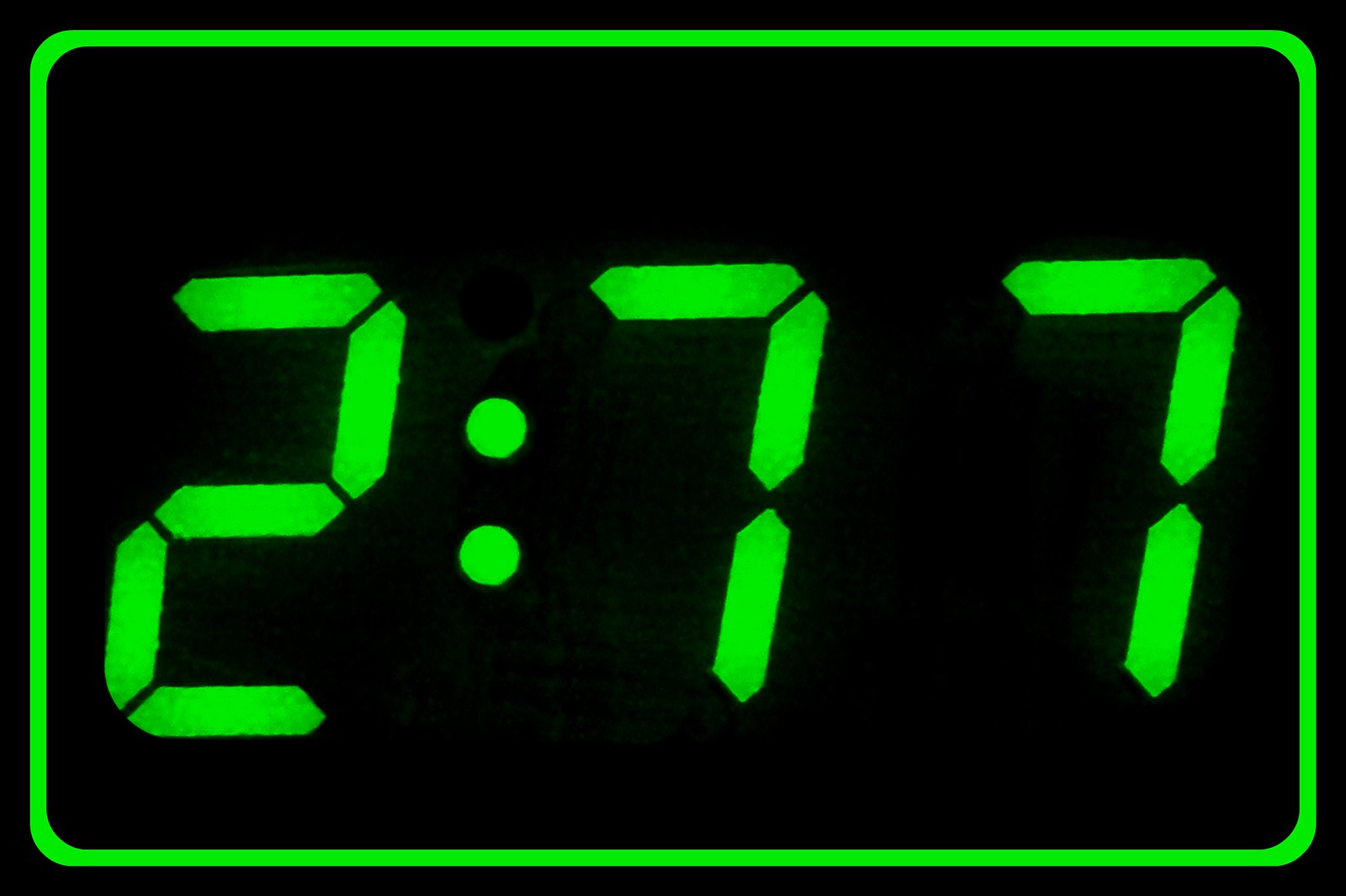This is an image showing what appears to be a digital clock screen. The screen is entirely black, with a bright, lime green display. The green display forms a large rectangle with rounded corners, and within this rectangle, there are digital numbers in a countdown or clock format. The numbers are unusually displayed as "2.77" using long hexagon shapes that resemble the style often seen on the television show "24". The green digits and border stand out vividly against the black background, giving it an unfamiliar and somewhat artistic appearance. The image overall suggests a modern digital clock, but the unconventional "2.77" reading adds a mysterious element, making it unclear what type of time or measurement is being represented.